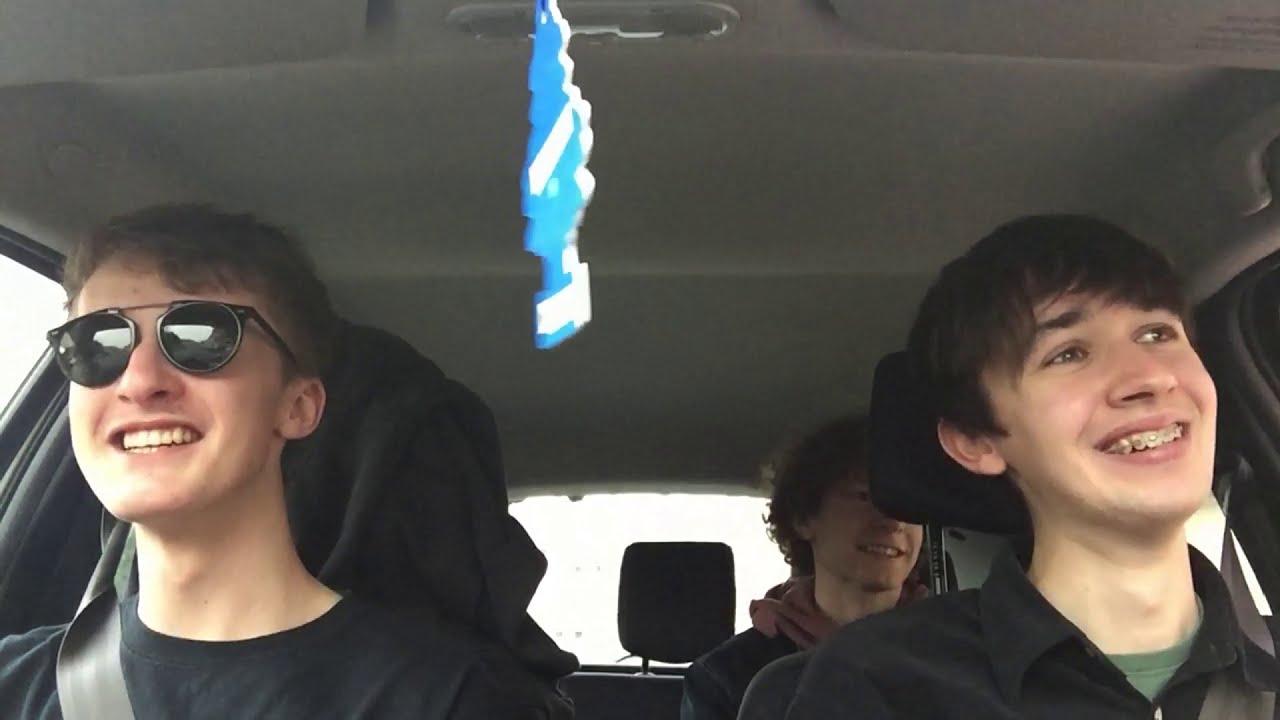In this image, three young boys are seen smiling in a car, suggesting a joyful moment among friends. The driver, who appears to be 16 or 17 years old, has short dark hair, braces, and is wearing a green t-shirt underneath a black collared jacket. To his left in the front passenger seat, another boy is wearing black sunglasses with a metal band across the lenses, a blue t-shirt, and there's a black jacket draped over the back of his seat. Both of them are securely fastened with gray seatbelts. In the back seat, positioned behind the driver, a third boy with long, curly hair and a hoodie can be seen. He also appears to be smiling, though his seatbelt is not clearly visible. Hanging from the rearview mirror at the top center of the image is a blue pine tree air freshener. The overall color palette includes shades of black, gray, blue, green, and brown, and the roof of the car is gray. The scene is likely captured during the day, highlighting a casual and cheerful car ride among friends.